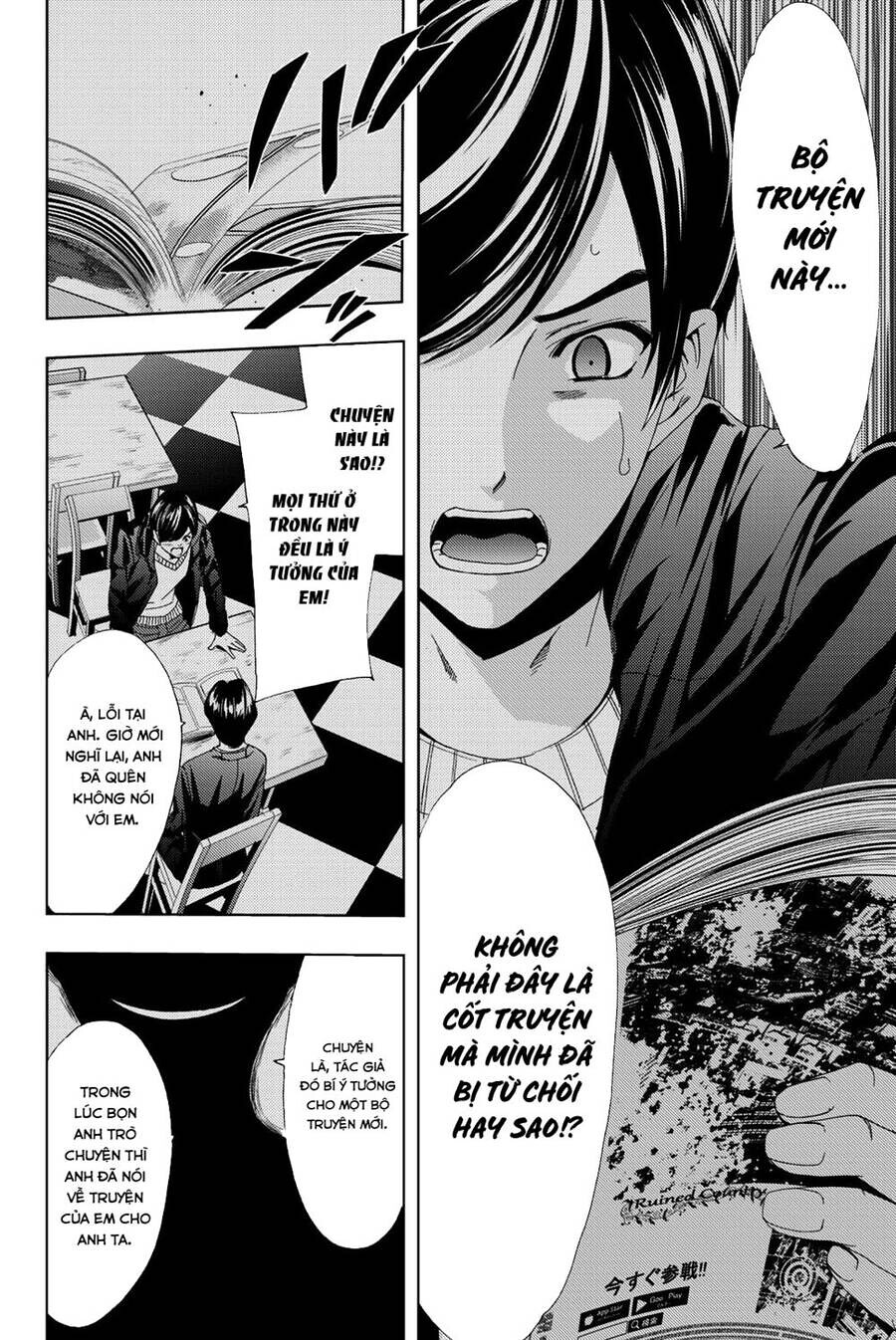The image captures a monochromatic page from a graphic novel or comic, with a clear, anime-style influence. On the right side of the page, a large vertical panel features a man weeping as he reads a book, his black, curved hair framing his open-mouth expression. This panel includes two black oval text boxes with italicized, non-English text.

To the left, there are three smaller, vertically aligned panels. The top panel depicts an open book from a side profile. The middle panel shows an overhead view of two boys in conversation; one is seated at a desk, focusing on the book before him, while the other stands opposite with his hands on the table, directing his gaze toward the first boy. The bottom panel is a minimalist black outline of a character with a speech bubble, expressing a smile.

Separating these panels is a white border, and the images themselves are overlaid with text and dashes, further contributing to the storytelling.